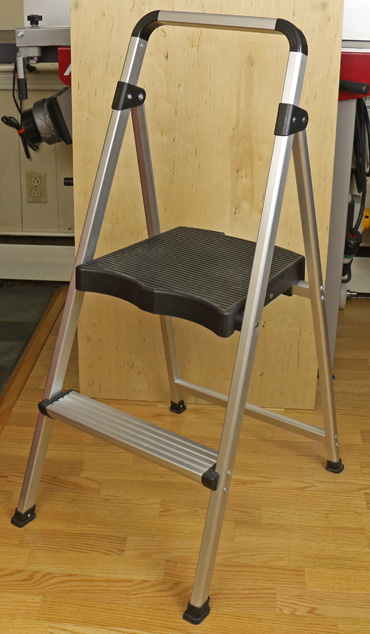In the image, a lightweight aluminum step stool with two steps is placed centrally on a light tan linoleum floor, which closely resembles hardwood. The stool features a smaller, lower silver step and a larger, upper step made of black hard plastic. The aluminum frame extends above the black platform with rounded corners at the top. The stool is positioned at a slight diagonal angle, giving a clear view of its structure.

The background consists of a light brown wooden wall. To the left, there is a motor attached to the wall, which looks like a hand sander with a circular top and a piece of sandpaper visible on its side. A light switch is also visible on the wall. On the right side of the image, a small red part is visible, possibly another tool. There is also a patch of carpet peeking into the image from the left. The image appears to be set in a workshop or a utility room. 

The colors in the image include shades of black, silver, tan, red, and gray, lending a utilitarian and functional aesthetic to the scene.